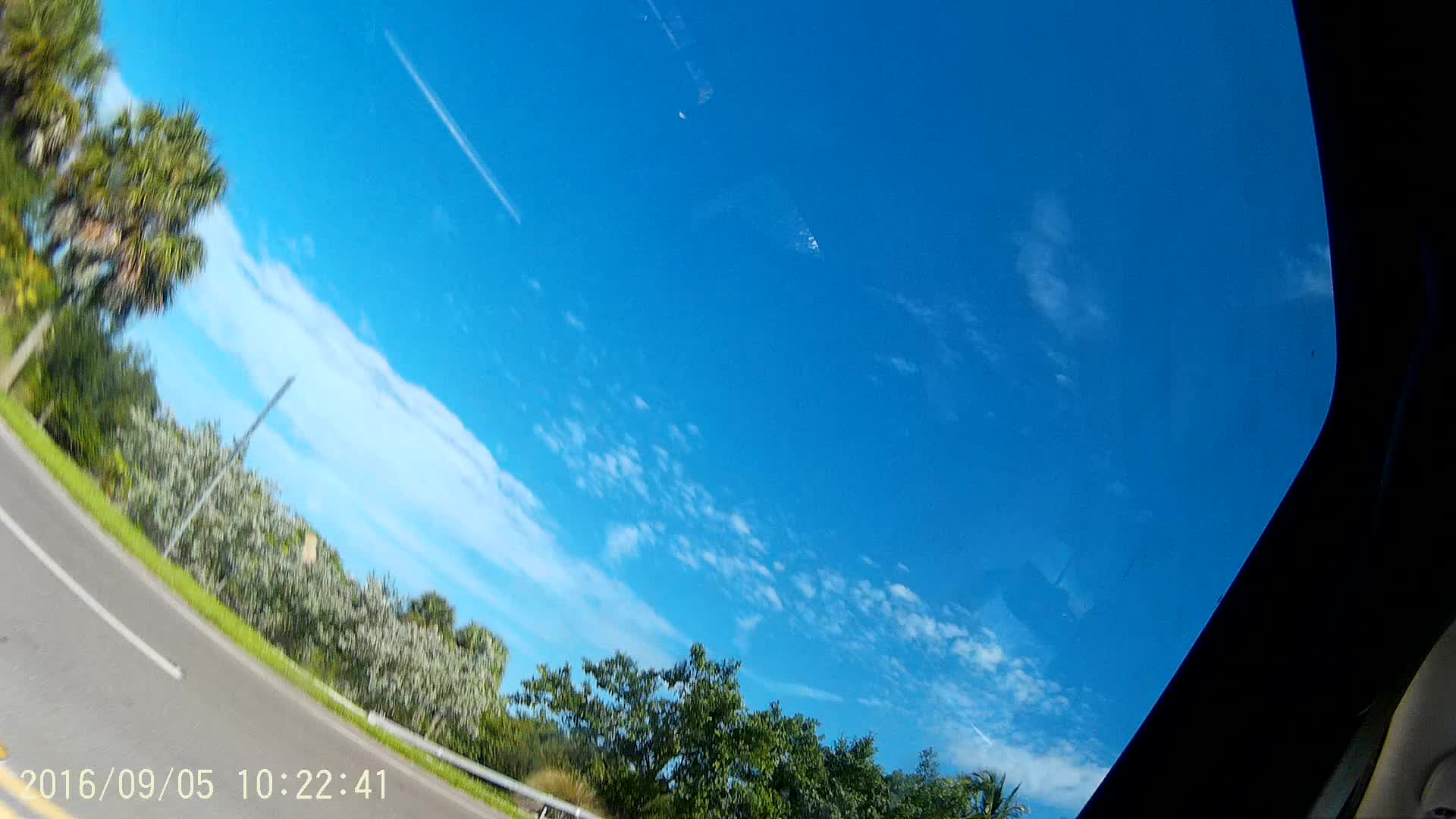This image captures a vibrant, sunny day seen from the interior of a vehicle, looking out through its windshield. The camera is angled slightly, creating a dynamic Dutch angle perspective. The clear blue sky is dotted with fluffy white clouds, indicating a bright daytime setting. Below the expansive sky, a stretch of gray asphalt road is visible, marked with white stripes and a partially cropped double yellow line. Alongside the road, lush green shrubs adorned with tiny white flowers add a touch of nature's beauty to the scene. A silver guardrail runs parallel to the road, ensuring safety. The black lining of the vehicle’s window frames this picturesque view. Notably, a timestamp reading "2016-09-05, September 5th, 10-22-41" is positioned at the bottom left, documenting the exact moment this serene landscape was captured.